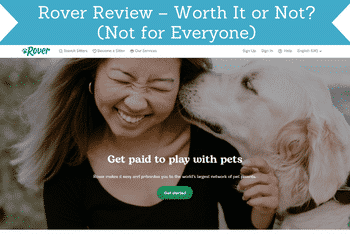The image is a small screenshot of the Rover website. A blue ribbon-like banner at the top center reads, "Rover Review: Worth It or Not (Not for Everyone)" in white text. Beneath this banner lies the screenshot of the website. At the very top of the website is a white horizontal bar with the word "Rover" in green on the left. To the right of "Rover" are small, clickable menu options, although their precise labels are hard to discern. On the far right side, there appear to be more clickable options likely related to signing up, accessing help, and selecting a language.

Below the navigation bar, there is a prominent image featuring a woman smiling as her dog licks her face. Superimposed on this image, there is a small piece of text that reads, "Get paid to play with pets." Directly beneath this text is a green button that seems to contain further instructions or a call-to-action, but the text is not entirely legible due to the small size of the image.